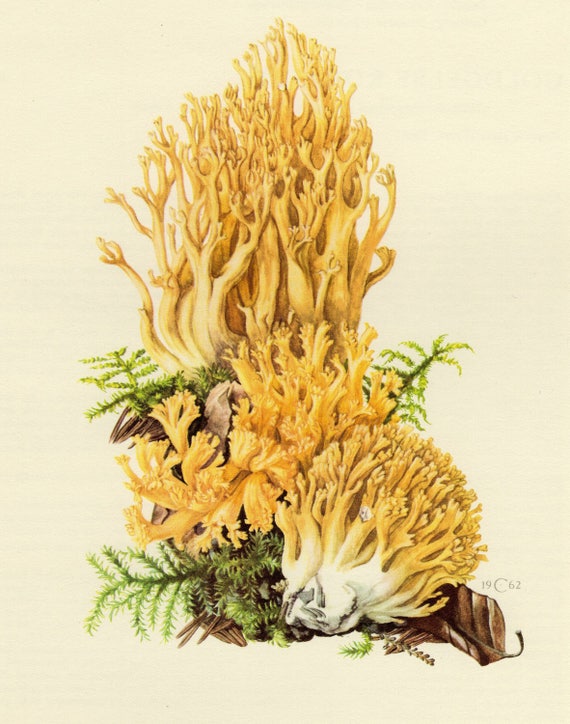The image is a rectangular color illustration of various fungi and natural elements, with the overall scene set against a tannish gray, almost cream-colored background. In the center of the drawing are three distinct yet similar types of fungi, each with white bases that transition into yellow tendrils. The fungi are arranged vertically:

- The bottom fungus emerges from a brown and green mixture of dead vegetation, including leaves and ferns. It's somewhat spherical in shape.
- The middle fungus also springs from a similar blend of dead vegetation, but its tendrils are thicker and more curved.
- The top fungus displays the longest tendrils, stretching upwards from the topmost part of a leaf, branch, and fern mixture.

These yellow tendrils extend substantially higher than those of the other fungi, creating a striking visual effect. Additionally, the image showcases various green leafy materials interspersed among the fungi, enhancing the naturalistic composition. Noteworthy details include the presence of some light brown elements in the center of the scene and the absence of any people or additional writing, except for the mark "19C62" located at the bottom right of the image.